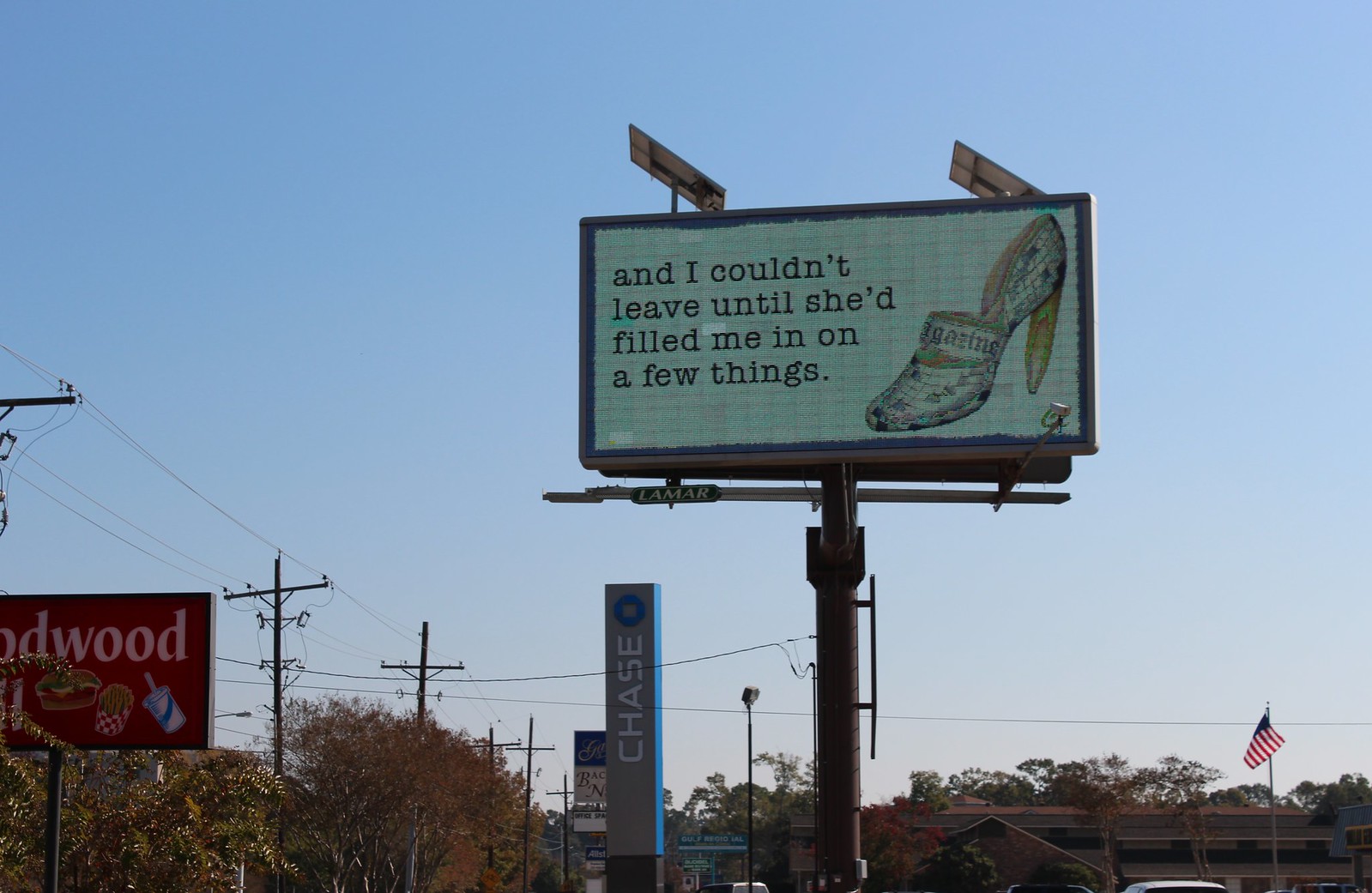The photograph captures a vibrant cityscape during a clear, sunny day. Dominating the scene is a several-stories-high billboard held up by a large cylindrical column. The billboard, framed in blue, displays a high-heeled shoe alongside the text, "and I couldn't leave until she'd filled me in on a few things." There is a noticeable light illuminating the billboard, emphasizing its prominence.

In the background, various other elements of urban life are visible. A red sign with drawings of a burger, fries, and a soda suggests the presence of a restaurant. Additionally, the Chase Bank sign stands tall on a gray column with the familiar blue circular logo at the top. The area seems bustling with modern infrastructure, as evidenced by the numerous electrical poles with overhead wires.

The lively atmosphere is complemented by an American flag billowing on a flagpole, indicating a gentle breeze. Trees in mid-color change add a touch of nature to the otherwise commercial setting. Lastly, the clear blue sky acts as a perfect backdrop, highlighting the dynamic energy of this urban environment.